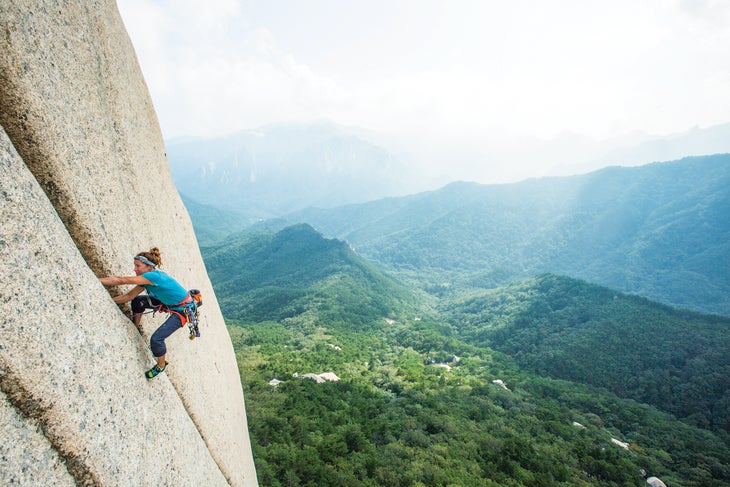In this vibrant outdoor photograph, a woman is seen rock climbing the imposing vertical face of a mountain on the left side of the image. The mountain's rugged surface is a mix of tan and brown hues with gray and black specks, featuring creases and gaps where she plants her hands to ascend. She is clad in a blue t-shirt and dark blue jeans, with a blue and black headband securing her hair. Her climbing gear includes an orange and black harness and a belt with various equipment such as ropes, chains, and hooks in yellow, blue, and white. Her climbing shoes are black with green tips and blue accents, complete with blue shoelaces.

To the right side of the image, a scenic valley unfolds, blanketed in lush, green trees and bushes, creating a picturesque contrast against the harsh rock face. The valley is uneven, featuring undulating terrain. The sky above is predominantly blue with white patches, indicating sunny weather. Distant mountains stretch out in various shades of green, and at the base, there are glimpses of tents or houses with white tops dispersed among the trees.